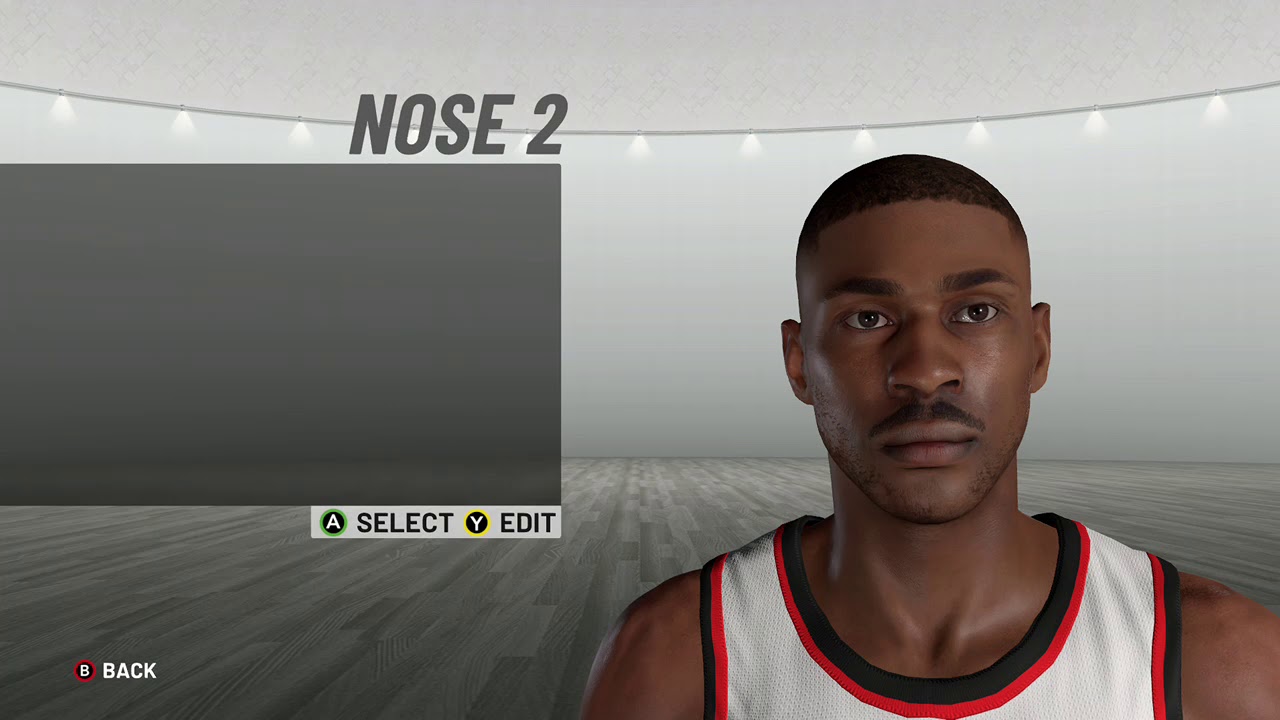This screenshot, captured from a video game, portrays an elegantly designed interior space as its background. The floor is composed of hardwood slats in various shades of grey, creating a patterned aesthetic with alternating dark and light tones. Stretching into the distance, the wall exhibits a gradient that transitions from a darker grey at the bottom to a lighter grey towards the top. A thin, curved line, medium grey in color, demarcates the wall from a barely textured light grey ceiling. This curved seam features downward pointing lights emitting white beams at consistent intervals.

Overlaying this background is the game's user interface. On the left, a dark grey rectangle hosts the text "Nose 2" in matching dark grey above it. Below this rectangle, a light grey box contains interactive buttons: a dark grey circle with a white "A" enclosed in green is labeled "Select," and next to it is a dark grey circle with a white "Y" encased in yellow, labeled "Edit." At the bottom left of the screen, another dark grey circle with a white "B," bordered in red, is accompanied by the word "Back" in white text.

Dominating the right side of the overlay, a basketball player emerges prominently. The athlete sports a white jersey, detailed with red and black trim around the neck and sleeves. The character is cropped just below the collarbones, emphasizing the upper torso and jersey design.